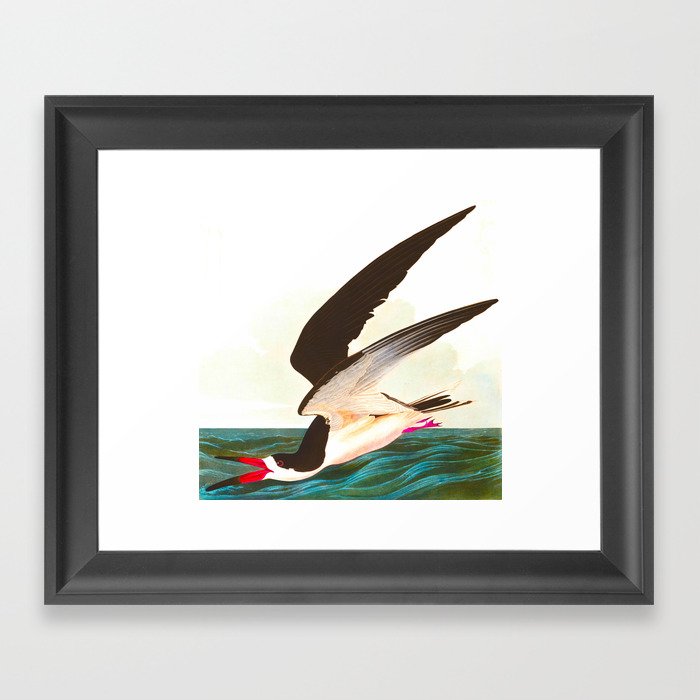The artwork, a stark piece depicting a bird, is framed in a black wooden frame and mounted against a light gray wall. The painting itself features a white background with the image of a distinctive ocean bird at the center. The bird has a dramatic posture, appearing to dive toward the abstract, greenish-textured ground below, which hints at water. The wings are expansive, painted black on top and white underneath, with the body showcasing a black upper half and a white underside. The bird's head is positioned on the ground with its beak open, displaying a red and black coloration. Its eyes are red, and its legs exhibit a pinkish hue. The detailed artwork captures the motion and intent of the bird, creating a vivid and lifelike depiction framed beautifully to highlight its striking contrast and dynamic composition.